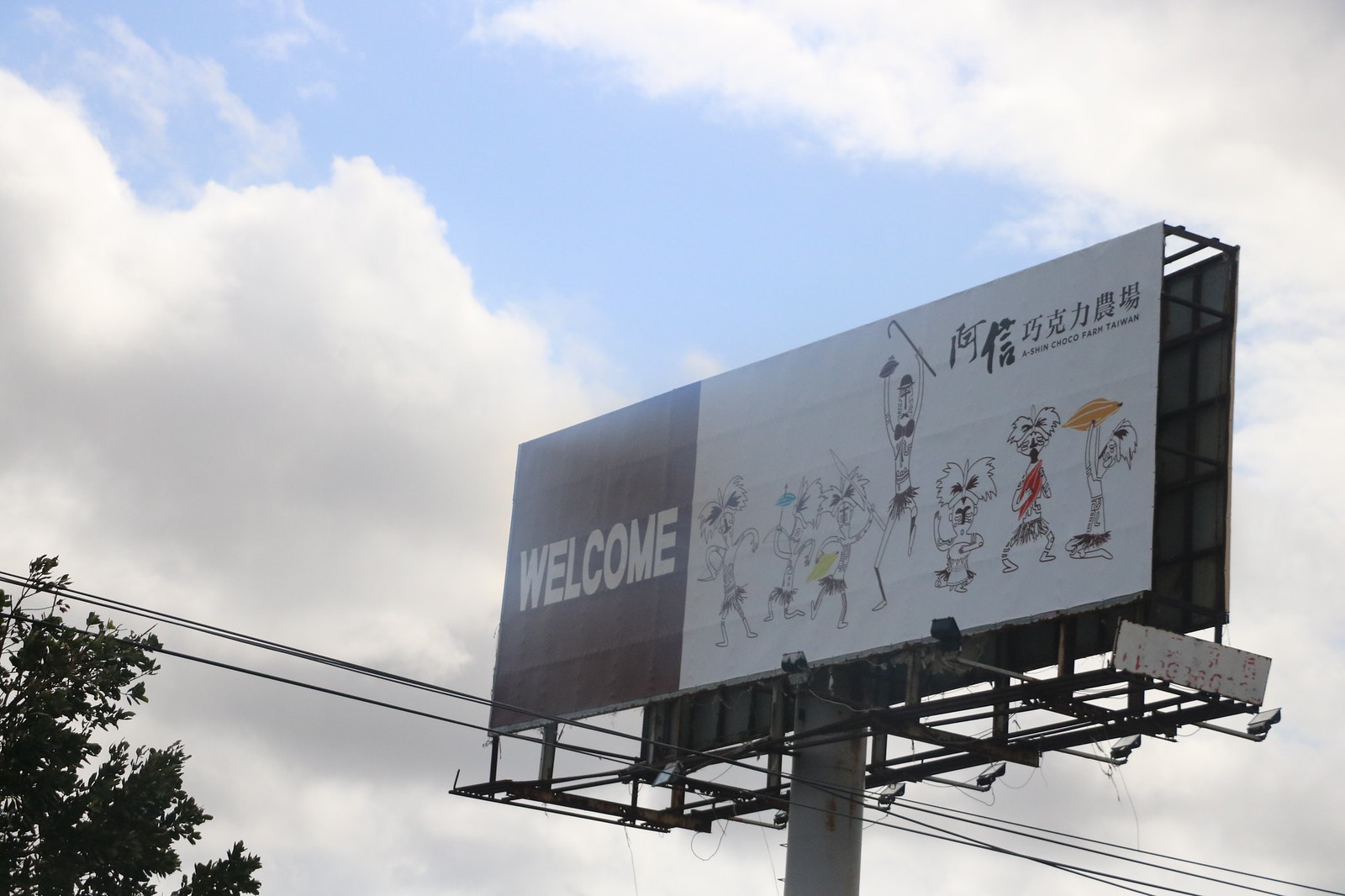The photograph features a large billboard standing tall against a predominantly cloudy blue sky, supported by a substantial, gray metal pole. The billboard's base is interwoven with several utility wires on the left side, appearing as though they nearly touch the framework beneath the sign. Below, on the left, the top of a tree is visible.

The billboard has a dark background. On the left side, "Welcome" is prominently displayed in white letters. The right side showcases a series of seven Asian characters, likely Japanese or Chinese, with one character distinctly taller than the others. Additionally, human-like, cartoonish figures are illustrated in black and white, appearing dynamic and playful, as if jumping and having fun. These figures are accented with vibrant shades of blue, yellow, red, and orange. The overall scene conveys a lively atmosphere amidst a serene backdrop of clouds and sky.